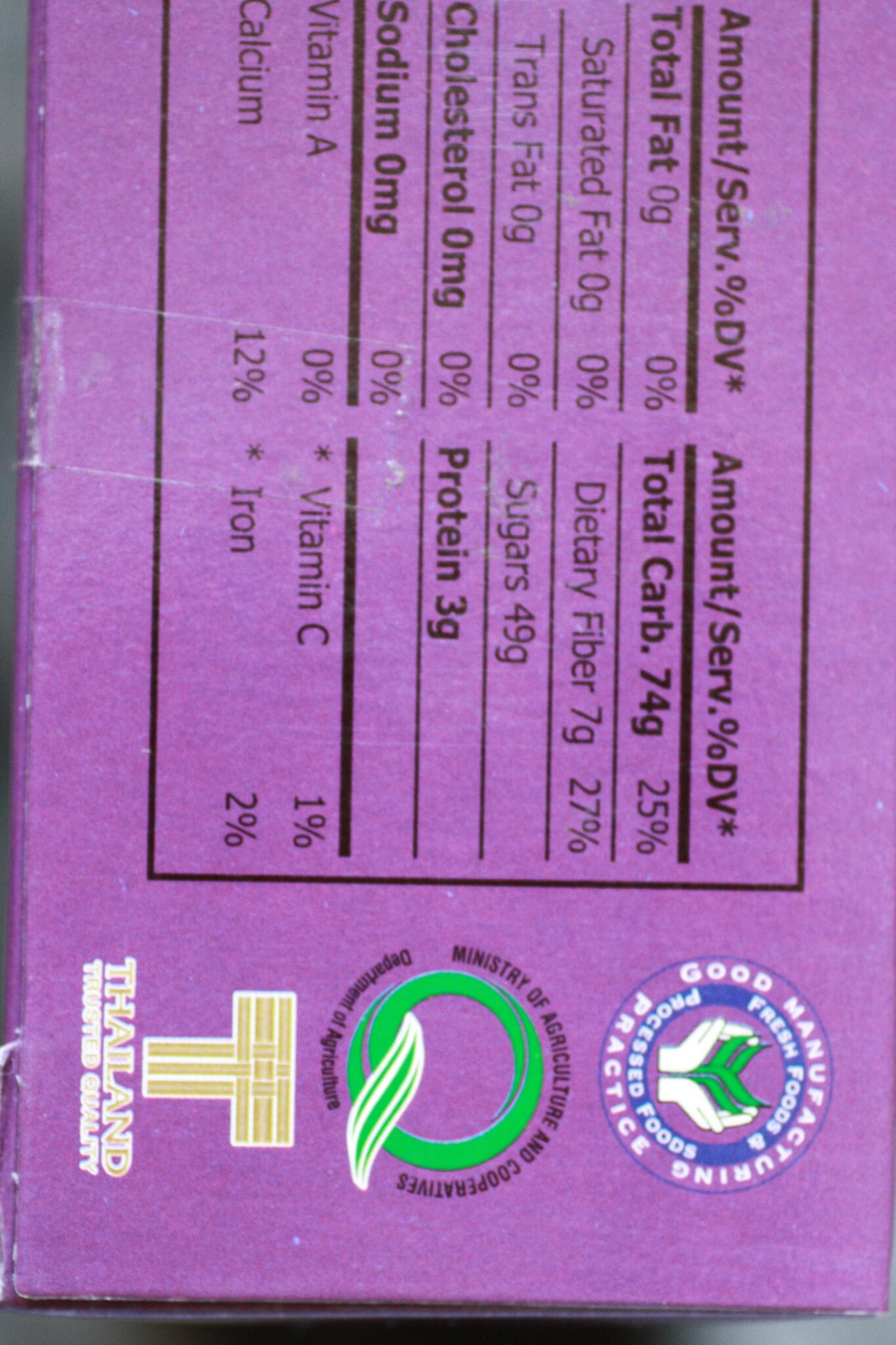Here is the detailed description of the food container label:

The food container features a purple label on the back, displaying nutritional information in a clear and organized manner. The label details the serving size, which provides specific nutritional values for the food product. Notably, the item contains 0 grams of total fat, constituting 0% of the daily value (DV). The total carbohydrate content is 74 grams, equating to 25% of the DV, with dietary fiber at 7 grams and sugars at 49 grams. Protein content is marked at 3 grams.

Vitamins and minerals are also listed, with Vitamin A at 0% DV, Vitamin C at 1% DV, Calcium at 12% DV, and Iron at 2% DV.

The product originates from Thailand and has been certified by the Ministry of Agriculture and Cooperatives, indicated by the presence of a Q logo on the label. This assurance of quality speaks to the standards upheld in the product's manufacturing and safety regulations.